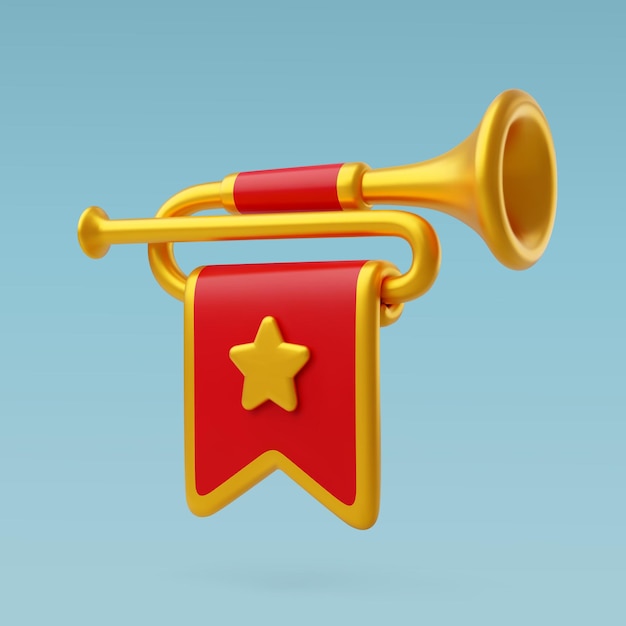This image is a cartoon-style, clip-art depiction of a royal bugle or trumpet-like horn, set against a baby blue background. The horn itself is a vibrant golden color and features a large bell facing to the right, with the mouthpiece on the left. The instrument has a complex structure, looping around itself with sections of pipe that go underneath and over the main portion.

A red flag with a gold trim prominently hangs from the lower part of the horn, and in the center of this flag is a perfectly centered golden star. The flag's vivid red contrasts with the golden hue of the horn, making for a striking visual effect. The image showcases different shades of gold, giving it a dynamic, sunlit appearance. There is no text or additional description within the image itself.